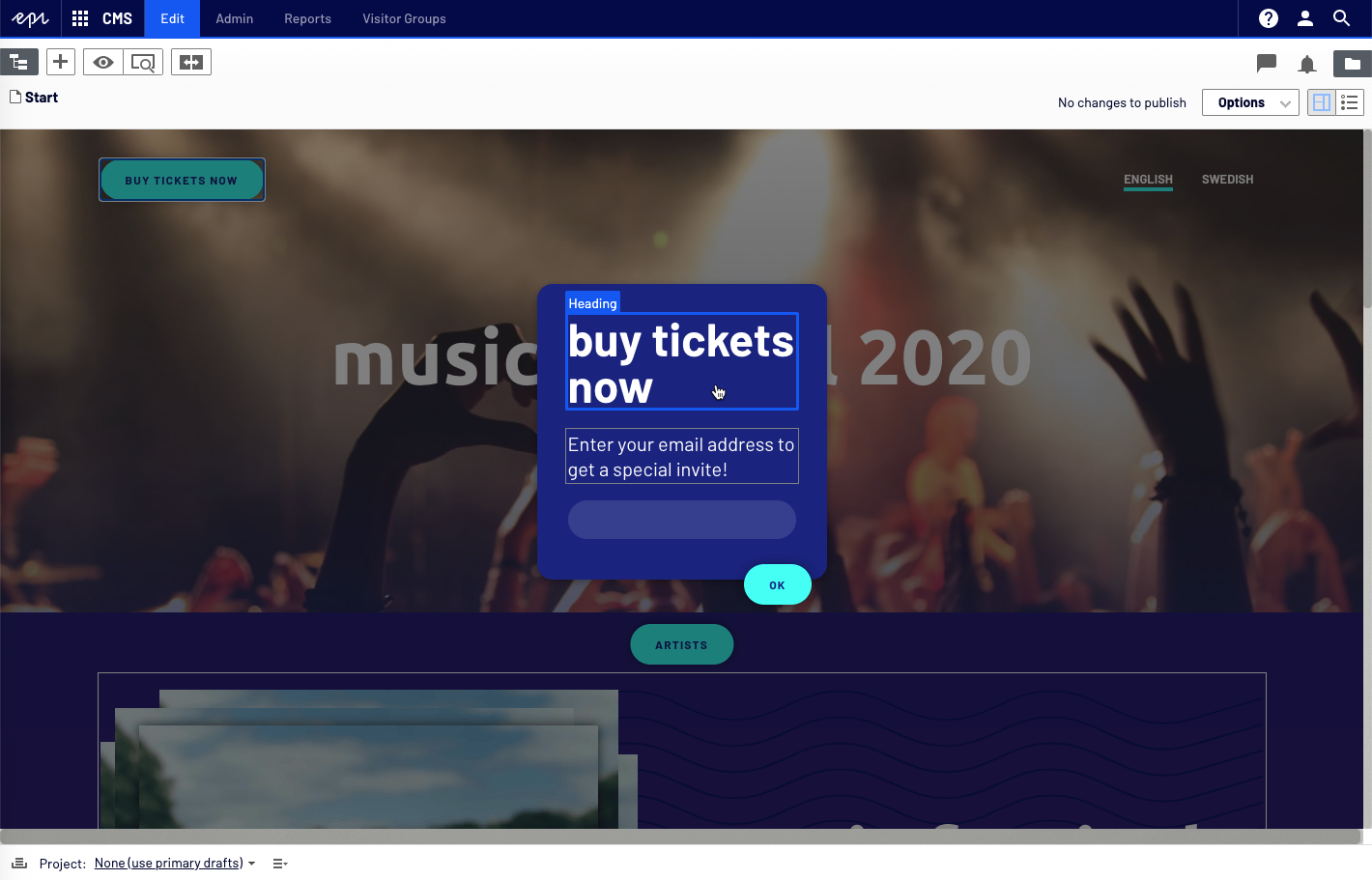The image showcases a music concert ticket purchasing website. Dominating the screen is a vibrant concert scene, presumably the main window of the site. Superimposed on this background, there is a prominent blue pop-up window with a bold heading in white font that reads, 'Buy Tickets Now.'

Inside the pop-up, the heading is set within a light blue square frame. Below this, there is a section inviting users to 'Enter your email address to get a special invite,' followed by a blank light blue bar where users can input their emails. At the bottom right corner of the pop-up, there is an 'OK' button in black font on a light green background, providing a clear call to action.